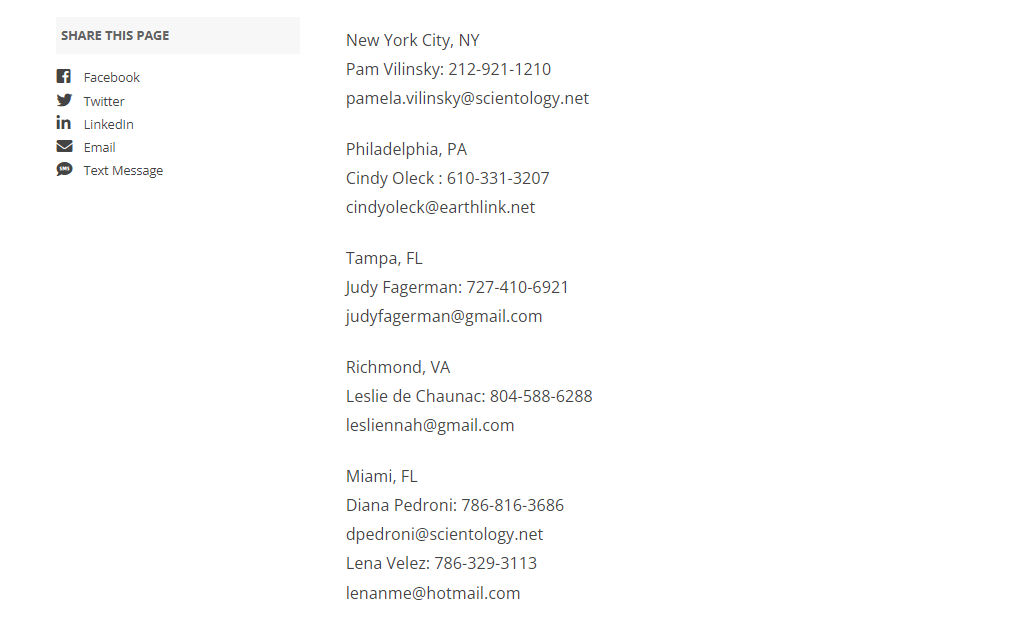The image features a text layout with two main sections, both written in black font. On the left side, there is a prominent option titled "Share this page," accompanied by various social media sharing handles. Each social media platform is represented with its respective grey icon: Facebook, Twitter, LinkedIn, email, and text message.

On the right side of the image, there is a detailed list of contact information for various individuals located in different cities. The text reads as follows:

- **New York City, NY**
   - Pam Vilinski: 212-921-1210
   - Email: Pamela.Vilinski@Scientology.net

- **Philadelphia**
   - Cindy Oleg: 610-331-3207
   - Email: Cindy.Oleg@Ethlink.net

- **Tampa, FL**
   - Judy Feigerman: 727-410-6921
   - Email: Judy.Feigerman@Gmail.com

- **Richmond, VA**
   - Leslie Da Chownak: 804-588-6288
   - Email: Leslie.Na@Gmail.com

- **Miami, FL**
   - Diana Petroni: 786-816-3686
   - Email: Dee.Petroni@Scientology.net
   - Lana Velez: 786-329-3113
   - Email: Lename@hotmail.com